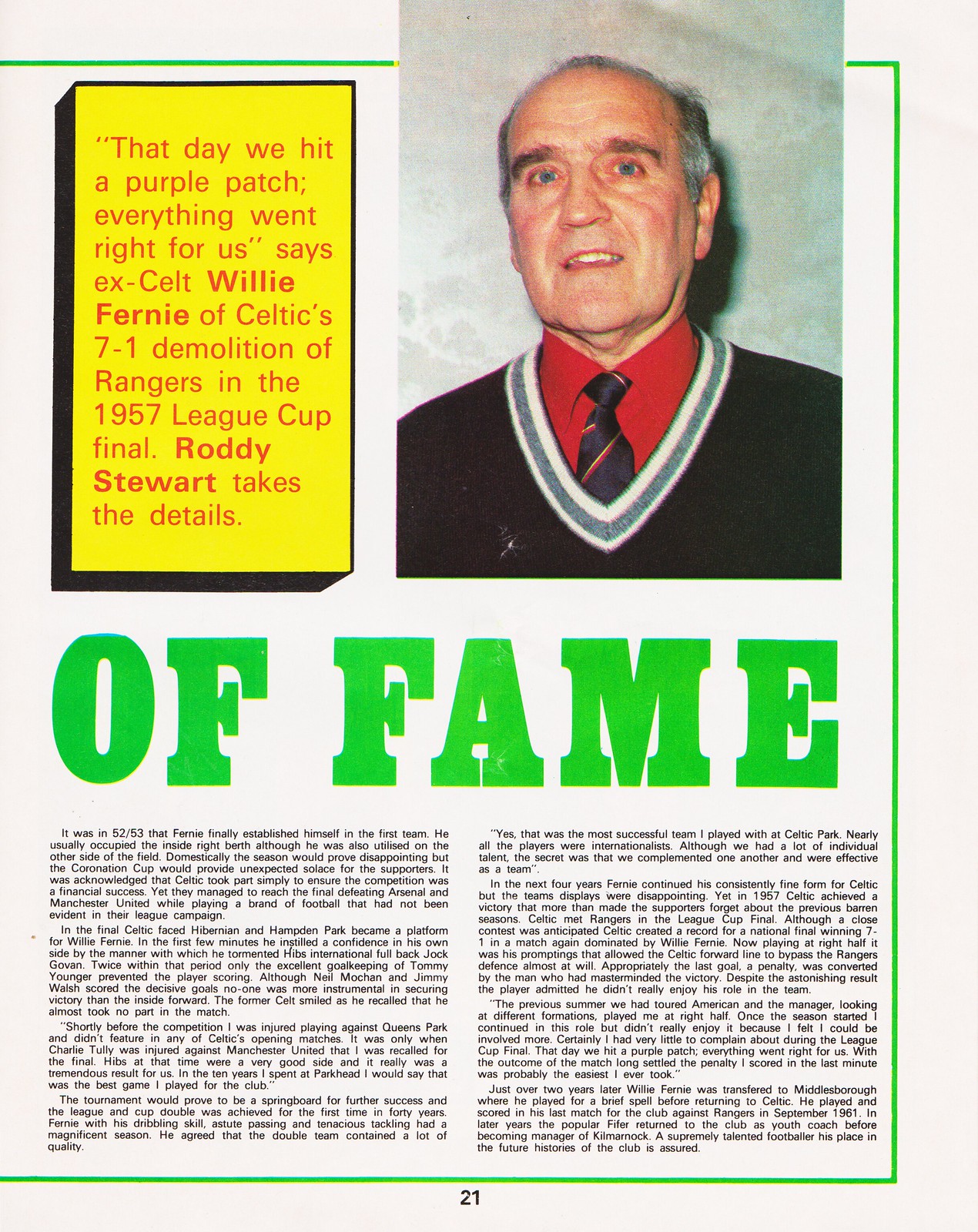This image depicts the right-hand page of a magazine, against a white or off-white background with a thin lime green border. At the bottom, it is labeled "page 21" in black text. In the top right corner of the page, there's a headshot of an older man, likely in his late 50s or early 60s, with blue eyes, partially balding grayish hair featuring darker streaks. He is dressed in a black V-neck sweater over a red button-up shirt and a black tie with red diagonal details. 

On the upper left, there is a prominent yellow box with a 3D appearance, containing a quotation in red text: "That day we hit a purple patch. Everything went right for us." This quote is attributed to ex-Celt Willie Ferny, referring to Celtic's 7-1 demolition of Rangers in the 1957 League Cup Final, with details accounted by Roddy Stewart.

Beneath the yellow box and the photograph, a bold title appears in lime green text reading, "Of Zane" (though the first word of this title is on the missing left-hand page). Below the title are two columns of small black text, presumably part of an article, although the print is too fine to discern.